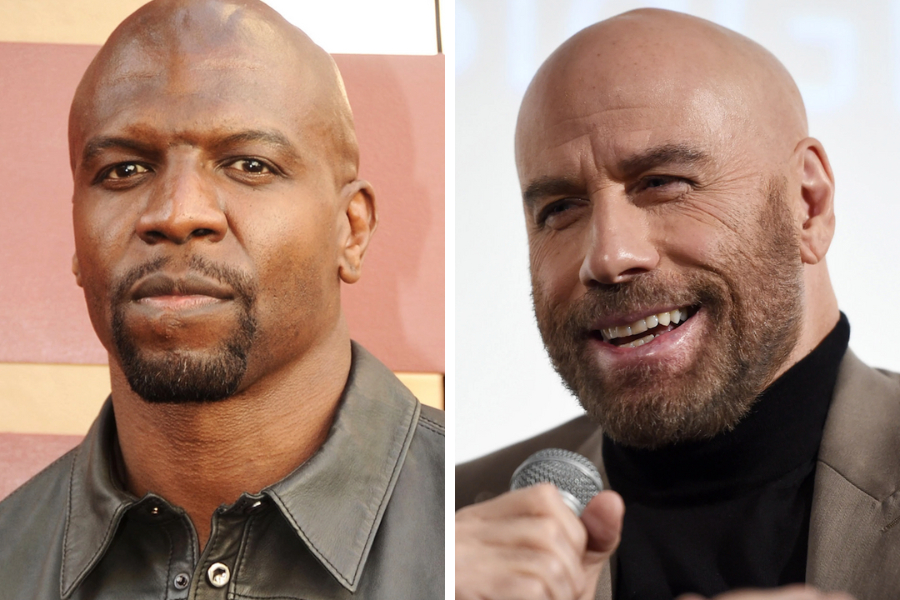The image features two close-up photographs of famous actors. On the left is a black man with medium brown skin, brown eyes, and a distinct facial hair pattern that includes a mustache area and a short beard along the bottom of his chin. He has a thicker neck and is wearing a black leather collared shirt. He looks intently straight at the camera. Though his exact identity is uncertain, he appears familiar and might be known from shows like "Brooklyn Nine-Nine" or "Reno 911!".

On the right is John Travolta, a well-known actor with tan skin, a bald head, and a dark brown beard. He is captured mid-laugh, with his eyes squinted and mouth open, showing his teeth. He holds a microphone in his hand and is dressed in a black turtleneck and suit. Both images exhibit headshots of the actors, highlighting their facial expressions and attire.